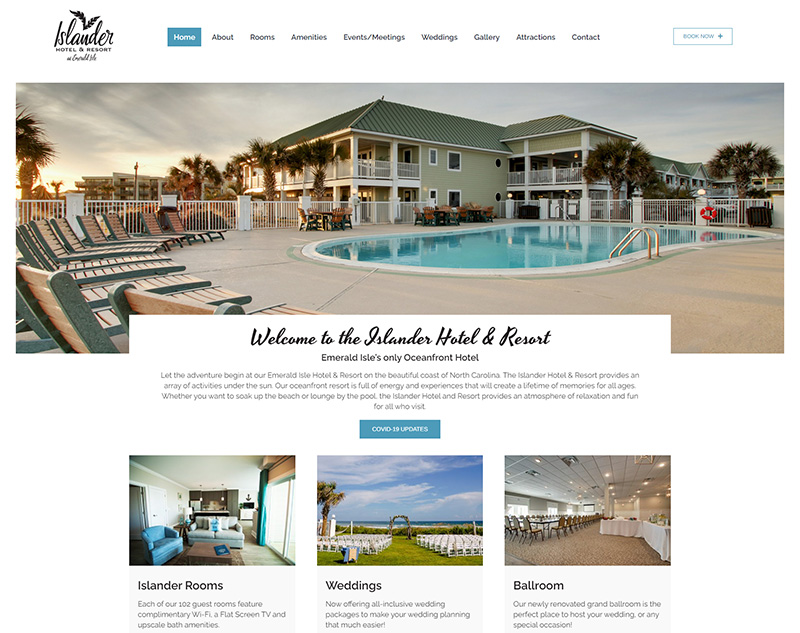Welcome to the Islander Hotel and Resort, Emerald Isle's only oceanfront hotel. Nestled on the picturesque coast of North Carolina, our resort promises the start of an unforgettable adventure. At the Islander Hotel and Resort, guests are treated to a myriad of sun-filled activities and experiences designed to create lifelong memories for visitors of all ages. Whether you choose to bask in the sun on the pristine beach or unwind by the pool, our resort offers the perfect blend of relaxation and fun. 

The resort's website features a blue button for COVID-19 updates, ensuring you stay informed about the latest health and safety measures. Below that, the "Islander Rooms" section showcases our beautifully appointed accommodations, furnished in calming green tones with comfortable couches and tasteful furniture.

The Islander Hotel and Resort also specializes in hosting weddings, set against the lush green lawns with neatly arranged chairs, providing a stunning backdrop for your special day. Additionally, our elegant ballroom, adorned with exquisite chandeliers, offers a sophisticated venue for receptions and other events. Experience the perfect getaway at the Islander Hotel and Resort, where every detail is designed to delight and impress.